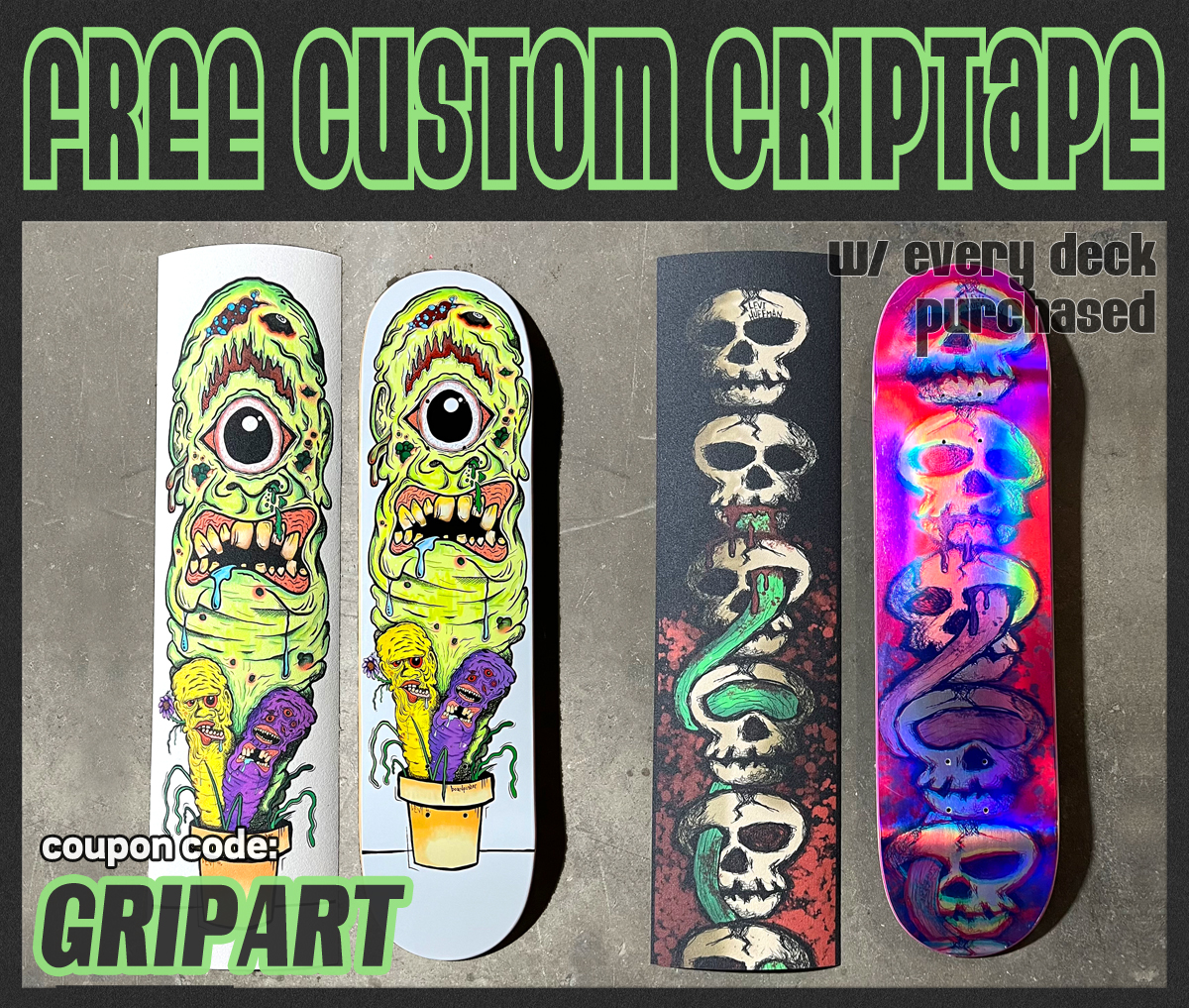The image features an advertisement for a custom design skateboard company, prominently displaying a black background with lime green-outlined text that reads "FREE CUSTOM GRIP TAPE with every deck purchased." The poster showcases four skateboards, each demonstrating unique custom grip tape designs. The two skateboards on the left present a grotesque and intriguing visual of a snotty, green cyclops creature emerging from a flower pot, with two smaller, equally grotesque monsters. This design is vivid with yellow crooked teeth, ooze dripping from the cyclops’ nose and mouth, and pustules on its forehead, all against a predominantly white background. On the right, the skateboards feature a more macabre theme, adorned with stacked skulls partially enveloped in blood-red hues. The skulls exhibit a snake intertwining through their eye sockets, creating a hauntingly detailed horror motif. Above these images, a note in green-lined black text directs viewers to use the coupon code "GRIP ART." The skateboards themselves range in style from standard rounded-end designs to more rectangular shapes, offering a diverse visual selection to potential buyers.